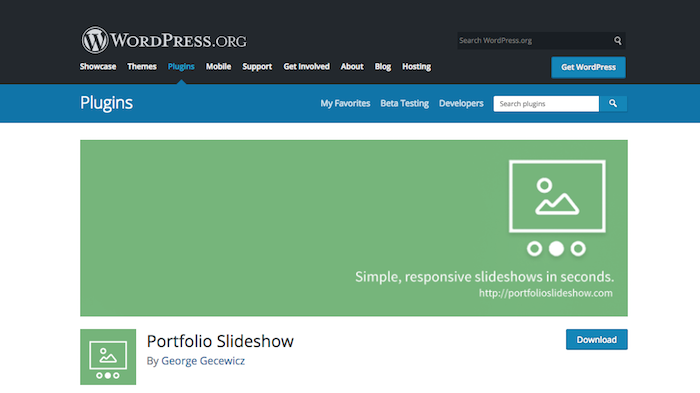The image captures a comprehensive view of the WordPress.org website interface, prominently showcasing its navigation menu and several key features. At the top, the navigation bar includes categories such as "Showcase," "Themes," "Plugins," "Support," "Get Involved," "About," "Blog," and "Hosting." Adjacent to these categories is a search field labeled "Search WordPress.org," allowing users to explore the site further.

Below this primary navigation, there are additional tabs focusing on "Showcase," "Product," "Plugins," "My Favorites," "Beta Testing," and "Developers," along with another search field specifically for plugins.

One highlighted section advertises a feature called "Simple Responsive Slideshows in Seconds," with a link to http://portfolioslideshow.com. This section includes a download button for the "Portfolio Slideshow" plugin, created by George Grewitch.

The color scheme of the website is visually striking, utilizing green, black, white, and blue elements to create a clean and professional look. This blend of colors enhances the readability and aesthetic appeal of the site, making the user experience both functional and visually engaging.